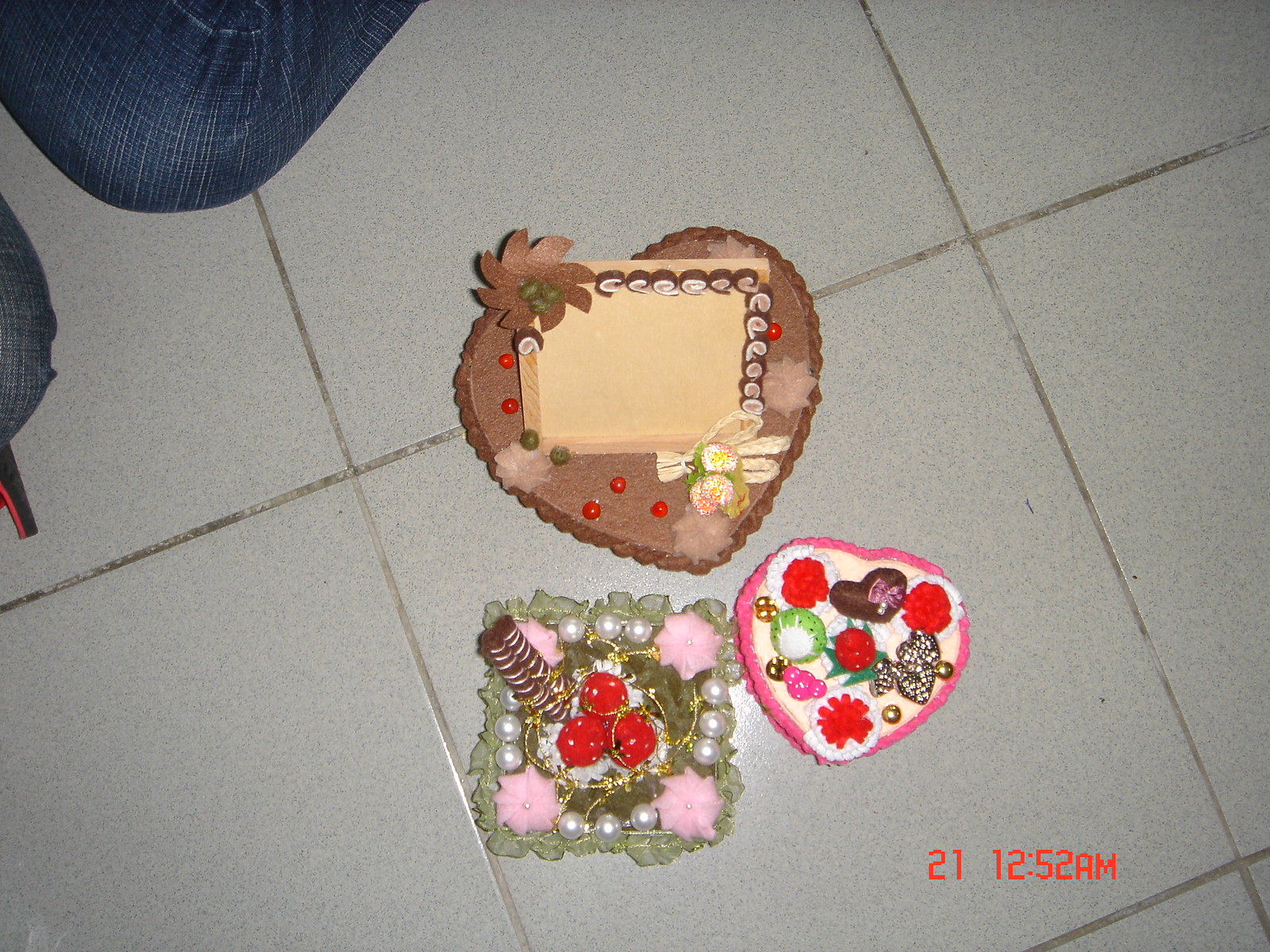The image depicts a delightful assortment of Valentine's Day-themed chocolate decorations, artfully arranged in a whimsical and engaging manner. These unique and intricate designs, likely intended as gifts, exude a fresh and fun vibe akin to offerings from a high-end candy or flower shop. The scene captures three main decorations placed on a surface where someone has taken a close-up photograph.

At the top of the image is a large, brown heart adorned with smaller candies, creating a striking centerpiece. To the left, there is a complex decoration featuring various shapes, enhanced with gold-colored string and beads, adding a touch of elegance and intricacy. On the right, another heart-shaped design is visible, also embellished with an array of candies, emphasizing the sweet theme of the occasion. In the bottom right corner of the image, the timestamp "12:52 a.m." suggests the photo was taken late at night, possibly after the recipient—perhaps a girl who received this from her boyfriend—decided to capture this special moment.